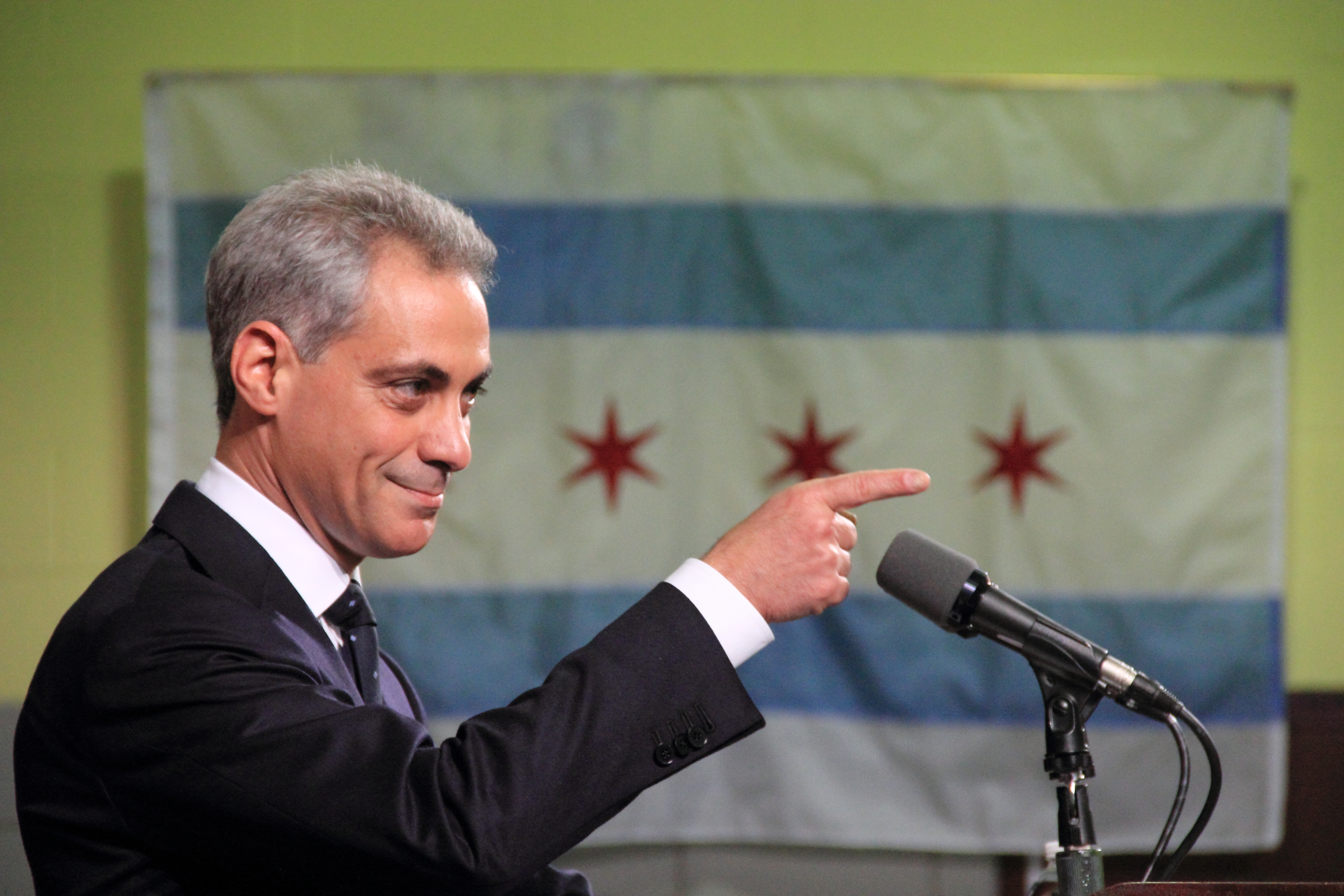This is a detailed photograph of a man who is likely a well-known politician, possibly Rahm Emanuel, speaking to a crowd. The man, who appears to be of Middle Eastern descent, has very short, salt-and-pepper hair and is slightly balding. He is wearing a black suit, a white button-down shirt, and a dark blue tie with light specks. He is pointing at the crowd with his right hand, his arm bent at the elbow, while smiling with his lips closed. In front of him, slightly to the right, there is a microphone. The background features a lime-green wall adorned with a recently unfolded flag. The flag has a horizontal pattern with white stripes at the top and bottom, blue stripes interspersed, and a central white stripe with three red stars.